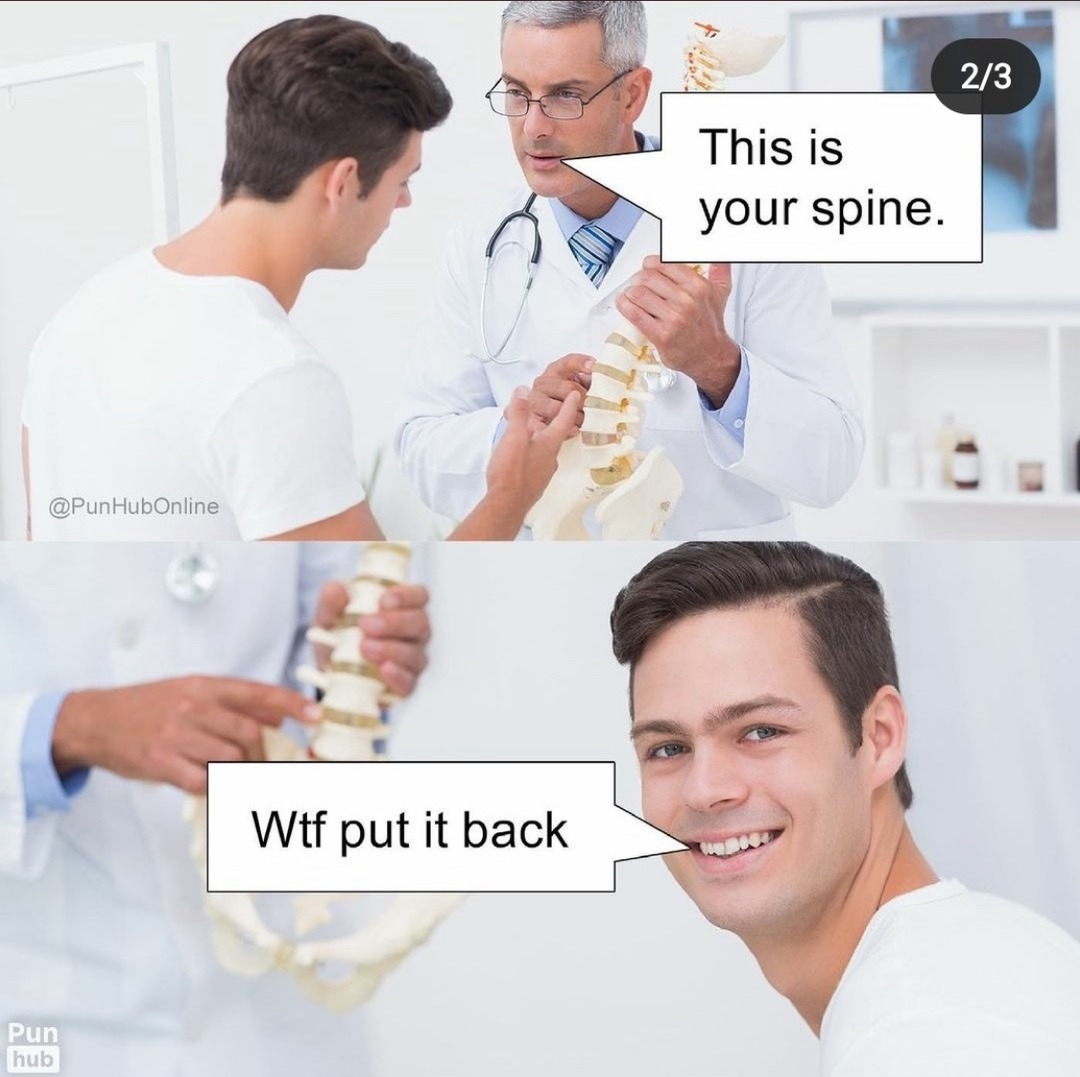In this two-part meme, the top half features a scene with a male doctor, distinguished by his gray hair, glasses, and stethoscope. He is holding a fake plastic model of a human spine attached to a hip, speaking to a white male patient with brown hair and dressed in a white t-shirt. A speech bubble with black text near the doctor's mouth reads, "This is your spine." In the bottom left corner of this top image, the credit "Pun Hub" is visible.

In the bottom half of the meme, the patient is now facing the camera directly with an expression of surprise. While only the doctor's torso is visible, he continues to hold the spine model. A speech bubble near the patient's mouth says, "WTF, put it back." The "Pun Hub" credit is again noted in the bottom left corner of this second image.